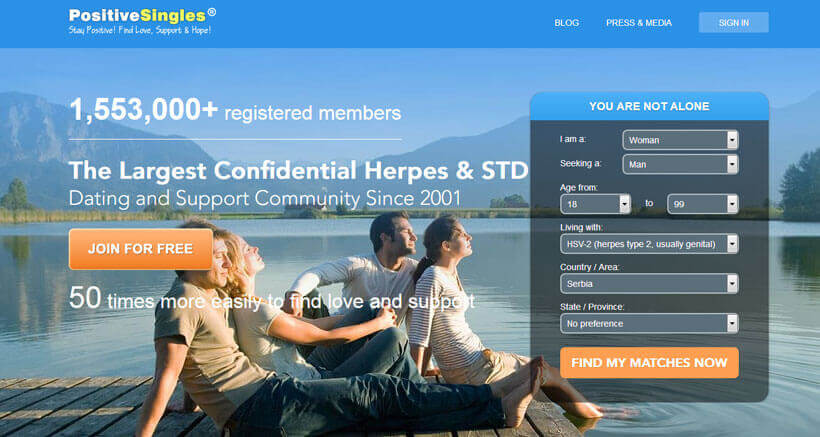In this website advertisement, the background features a serene scene with picturesque mountains beyond a tranquil lake. In the foreground, four individuals are seated on a dock, enjoying the peaceful setting. The group includes two men and two women. One man wears a tan shirt paired with blue jeans and is barefoot. The second man dons a white long-sleeve shirt, while his pants remain unseen as they are partially covered. Sitting beside the man in the tan shirt, a blonde woman sports a white shirt and blue jeans. The other woman, who has brown hair, is dressed in a white and gray striped shirt and tan capri-style pants, with her legs dipped in the water.

The image predominantly features blue hues, contributing to the calming atmosphere. In the top left corner of the page, a light blue header displays the words "Positive Singles" with additional text underneath it. To the right in the header, white text lists "Blog," "Press and Media," and "Sign In," the latter within a small square box.

Prominently overlaid on the middle of the page, above the scenic background, it reads: "1,553,000+ registered members. The largest confidential herpes and STD dating and support community since 2001." Below this, there's an orange clickable button labeled "Join for Free."

To the right, the text reassures users with "You are not alone," followed by fields for personal details and an orange button at the bottom marked "Find My Matches Now."